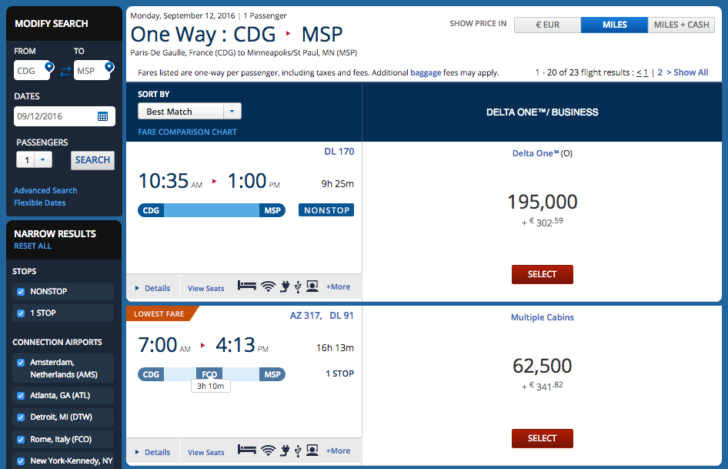A detailed screenshot of a flight booking webpage features a clean white and blue color scheme. The interface displays search criteria indicating the user is looking to book a flight from France to Minneapolis, scheduled for Monday, September 12th, 2016. On the left side of the page, a sidebar contains a small box with search parameters including dates, departure and arrival locations, and the number of passengers. Beneath this box is another section with additional filters such as preferred flight types and the number of stops, allowing the user to refine their search results.

Dominating the right-hand side is a large white results window detailing the available flights. The results prominently display the travel itinerary from Charles de Gaulle Airport (CDG) in Paris to Minneapolis–Saint Paul International Airport (MSP). At the top, there is a 'Sort by' option offering different sorting criteria. Two flight options from Delta Air Lines are presented. 

The first option shows a non-stop flight departing at 10:35 AM and arriving at 1:00 PM, totaling 9 hours and 25 minutes. 

The second option lists a flight departing at 7:00 AM, featuring one stop, and arriving at 4:13 PM, with a total travel time of 16 hours and 13 minutes. Additionally, details regarding points accumulation are displayed, likely indicating the number of points required for booking, pertinent to Delta One members.